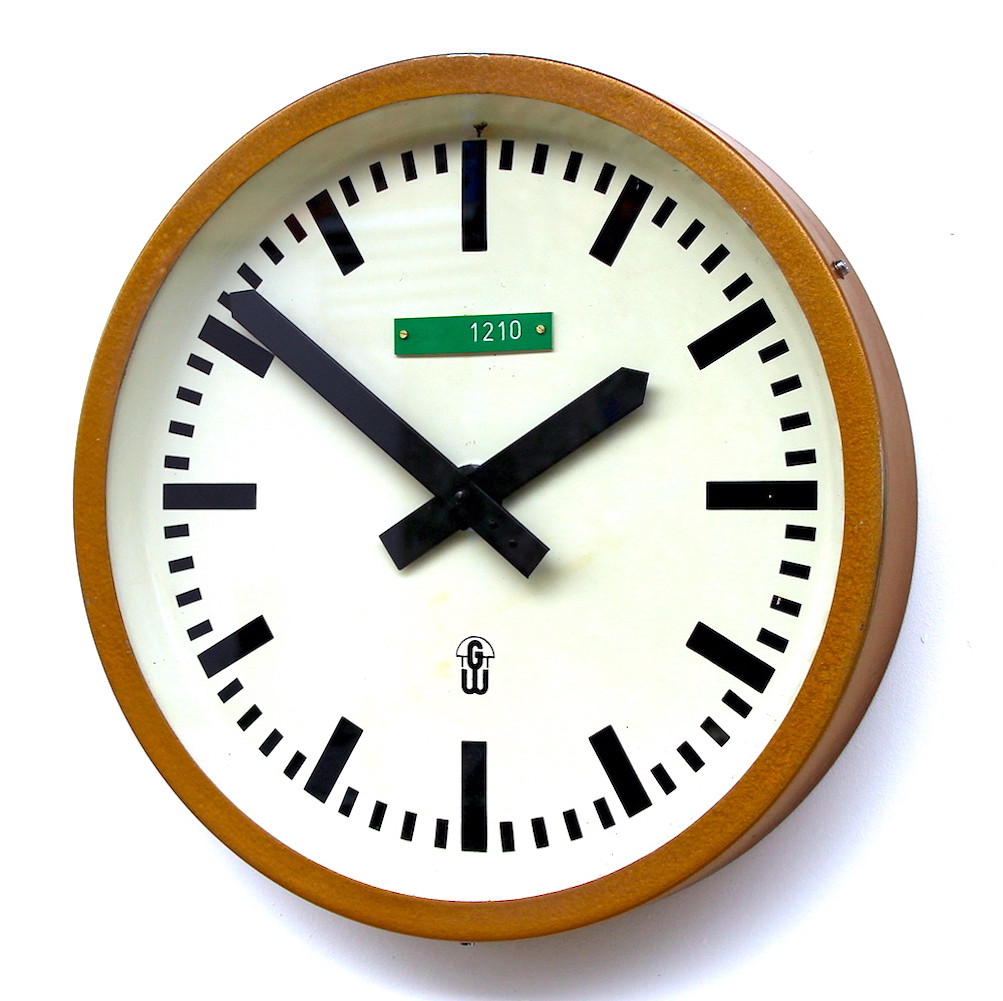Here is the cleaned-up and detailed caption for the image:

"This image features a clock prominently displayed against a plain backdrop, devoid of any background elements. The clock face is pristine white, bordered by a stylish bronze frame. Notably minimalist, the clock lacks numerical markers, instead having simple black lines to indicate the positions where the numbers would traditionally appear. Below the 12 o'clock line, there is a distinctive green metal tag, square in shape, inscribed with the number '1210' in white. The clock's time reads 2:51, as indicated by its black hour and minute hands."